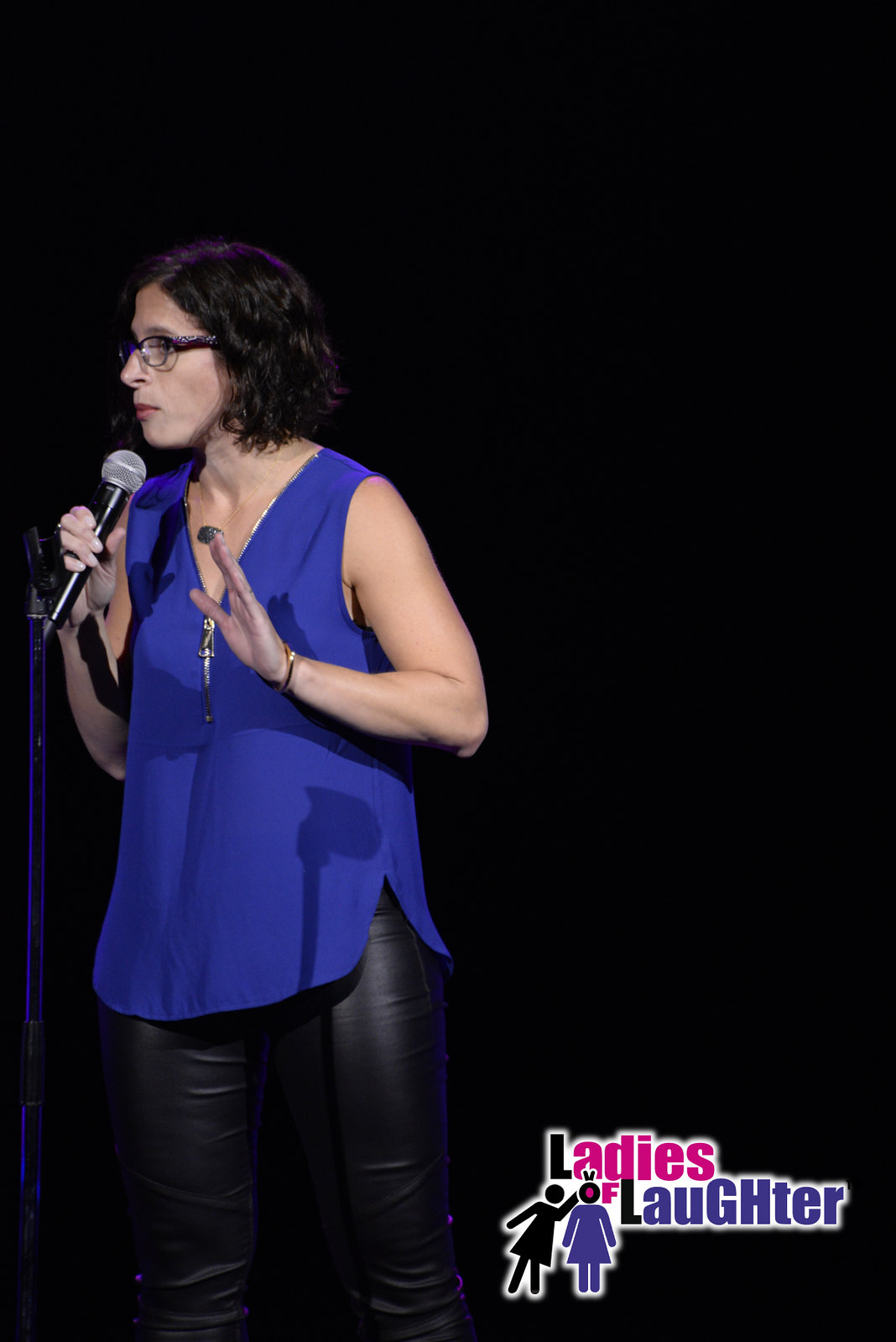The image features a woman with short black hair and eyeglasses, standing on the left side against a completely black background. She is wearing black leather pants and a dark blue, zippered tank top. In her right hand, she holds a black and silver microphone up to her face, while her left hand is raised, palm facing up, as if addressing an audience. A gold bracelet adorns her left wrist. At the bottom right corner of the image, pink and blue text reads "Ladies of Laughter." Additionally, there's a silhouette of two women: one in a black dress with fingers raised in a playful gesture above the head of a second woman in blue, akin to restroom sign figures. The scene appears to capture a moment of animated public speaking or performance.